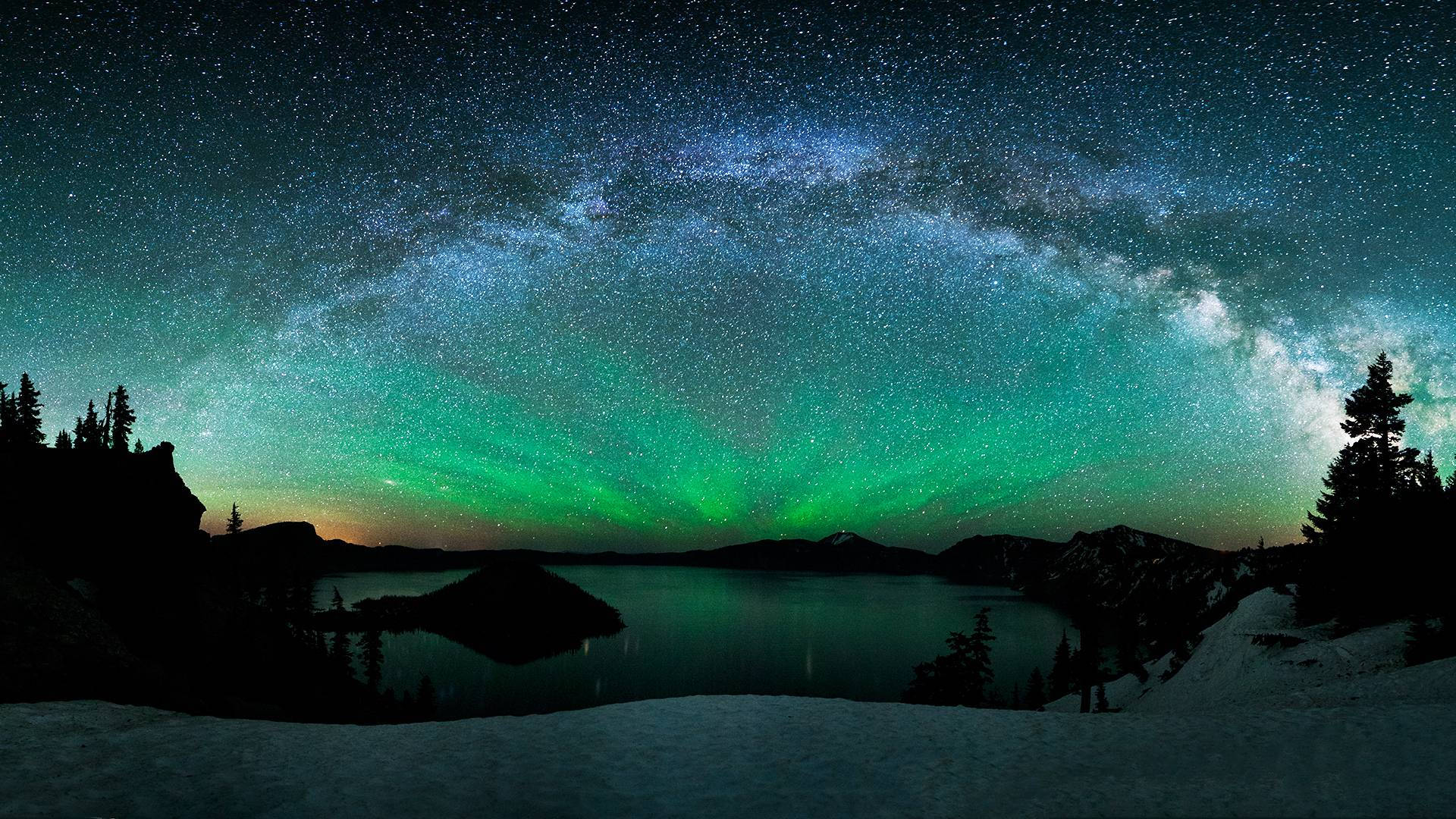This is a panoramic color photograph capturing a stunning nightscape atop a large, snow-covered mountain. The foreground displays the pristine white snow, while silhouetted pine trees add a natural frame to the scene. The skyline is dominated by the expansive, star-filled night sky, with a particularly detailed depiction of the Milky Way stretching across the image. 

A setting sun is just visible to the left, casting a faint glow upon the landscape. Beneath the starry sky, vibrant aurora lights in shades of green, purple, and blue streak across the horizon, adding a magical touch to the photograph. 

Mid-ground features include a dark lake, barely visible except for the silhouette of a small island. To the left of the lake, there appears to be the dark outline of a building, possibly a house with a dock extending towards the water, adding a sense of human presence to the otherwise wild and natural scene.

Overall, the photograph beautifully captures the serene and mesmerizing beauty of a winter night, where the celestial and earthly elements combine harmoniously.